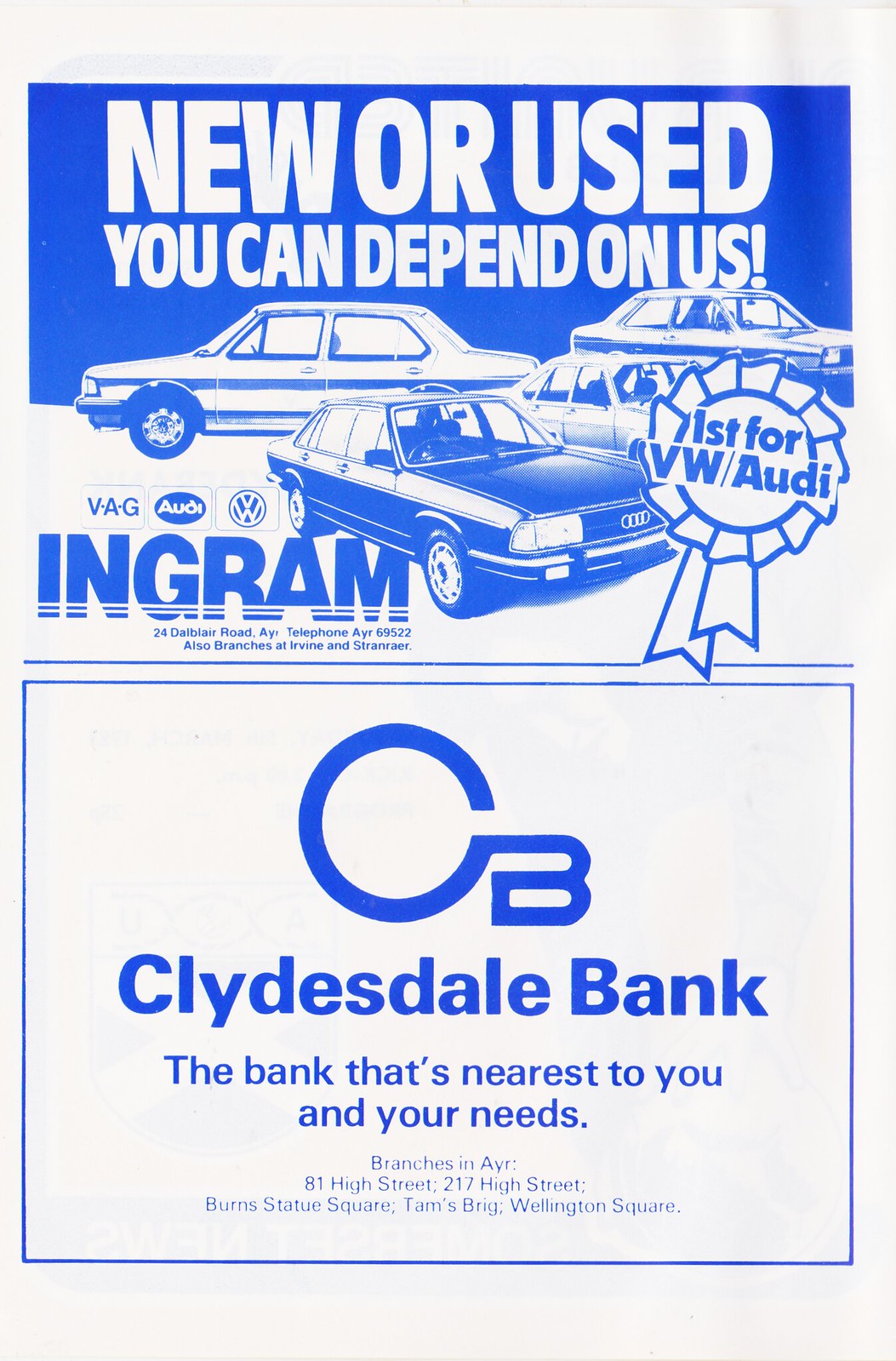The image displays a bifurcated poster predominantly in blue and white tones, featuring advertisements both at the top and bottom. The top section showcases an ad with a blue background occupying the upper third, prominently displaying the tagline "New or Used, You Can Depend on Us" in white font. Below this, a stylized illustration of four cars is presented—three in a blue and white monochrome scheme, and one in full blue—arranged with varying orientations; one car faces left, another is angled towards the front right, and the remaining two are aligned towards the lower right corner. This section also features brand logos and text: "VAG", "Audi", and the "Volkswagen" emblem, accompanied by the name "Ingram" in large print positioned vertically along the left side, and a ribbon graphic on the right stating "First for VW/Audi". An additional detailed address, "24 Del Blair Road, AY, telephone AYR 69522, with branches in Ayr, Burnside, and Newton," is provided.

The bottom section features an ad for "CB Clydesdale Bank," accompanied by the tagline "The bank that's nearest to you and your needs," followed by the specific address, "Branches in AYR: 81 High Street, 217 High Street, Burns Statue Square, Thames Brigg, Wellington Square."

This elaborate composition merges details from the voices, emphasizing the visual elements and textual information central to the advertisement.